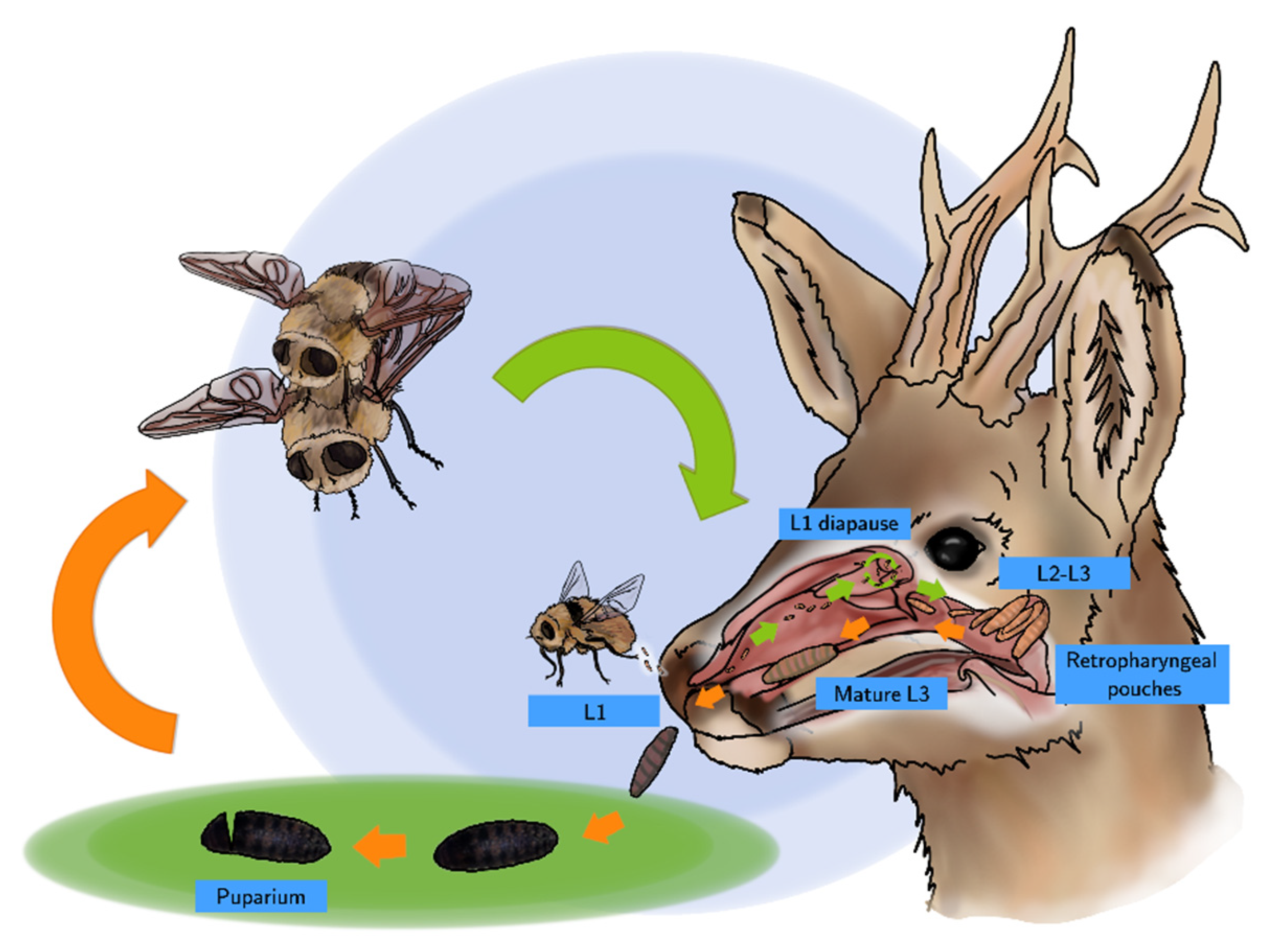The infographic illustrates the reproductive cycle of a parasitic fly using a deer as its host. The background features concentric light and darker blue circles. On the right side of the diagram, the focus is on the head of a brown deer, detailed with large antlers and upright ears. The deer's nasal passage and mouth are dissected to reveal the internal process of parasite infestation. Green and orange arrows depict the movement of the fly larvae. Initially, one fly deposits its larvae into the deer's nose. These larvae, labeled L1 diapause, L2, and L3 stages, develop within the nasal passage and retrofarnageal pouches before maturing to L3. The mature larvae then exit through the deer's mouth, drop to the ground entering the puparium stage, and finally emerge as fully-grown flies.

In the top left corner, two mating flies—brown with black eyes and tails—are shown. Below them, another fly deposits larvae into the deer's nose. The lifecycle completes as illustrated by green arrows pointing towards the deer's nasal passage and orange arrows circling back to the mating flies, emphasizing the cyclical nature of this parasitic relationship. Detailed inset images depict the larvae exiting the deer's mouth, transforming on the ground, and hatching from their pupae.